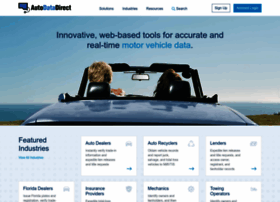Screenshot of a website displayed on a white background. The image itself is quite small. Prominently featured is a keyboard with the words "AUTO" in black, "DATA" in blue, and "DIRECT" again in black. At the center, there are four blue words that are unreadable. On the far right, there's a white rectangle with blue text and next to it, a blue rectangle with white text, both of which are illegible. 

Below this, there's an image that looks like generic stock footage of someone driving down a road with a blue background and darker blue text that reads, "Innovative web-based tools for accurate and real-time." Below this, in light blue text, it says, "motor vehicle data." In the background, there's a blue convertible with the top down; a man with blondish hair is driving, and a woman with brown hair is sitting in the passenger seat. Scattered across the image are additional white text boxes filled with blue text, though the content of these boxes is unclear. 

The caption also notes that there have been some issues with the website that are in the process of being resolved.